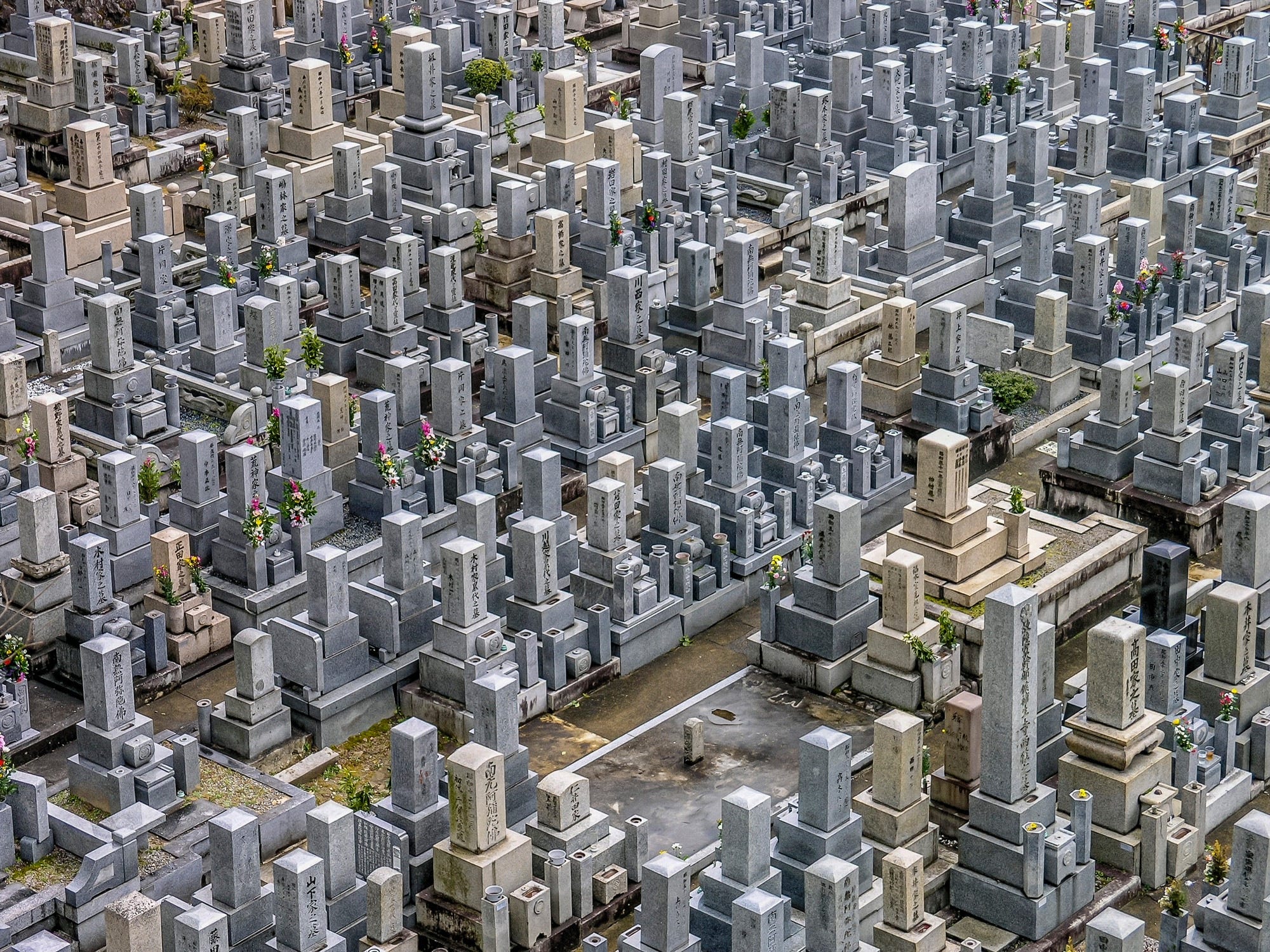This aerial photograph captures an extensive and meticulously organized cemetery, likely situated in either China or Japan. The graveyard is densely packed with numerous grave markers, each composed of stacked rectangular concrete blocks, forming towering structures. These markers predominantly display inscriptions in Asian scripts, most likely kanji. The tombstones, varying in shades of gray and tan, are arranged in extremely straight rows, creating very narrow walking paths between them.

Among the markers, some feature small vases with pink and white flowers, while others have torches that appear to be lit. There are concrete pillars and occasional small bushes interspersed throughout the area. Moss and mildew cover some of the older markers, offering a stark contrast to the cleaner, more modern ones.

The image reveals a vast number of graves, suggesting a potential count in the thousands, although at least a hundred are clearly visible. Some headstones are elevated on platforms, indicating possibly larger or family plots. The overall scene is an almost monochromatic expanse that one might initially mistake for a cityscape, reflecting the overwhelming number of tombstones and the close proximity in which they are placed.